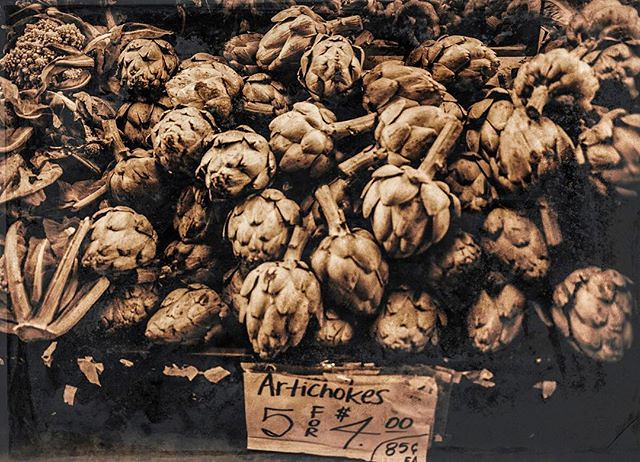This sepia-toned photograph captures a rustic display of numerous artichokes stacked atop each other on a worn black platform, which appears to be a table or a bin with remnants of previously taped signs. The artichokes, with their heads facing forward and stems pointing away, dominate the frame, creating an abundance that extends to the photograph's edges. A handwritten sign, crafted from brown paper, prominently reads, "Artichokes - Five for $4.00 or 85 cents each," in black marker. The sepia filter lends a nostalgic golden hue to the scene, emphasizing the deep shadows and rich textures of the artichokes and their setting.